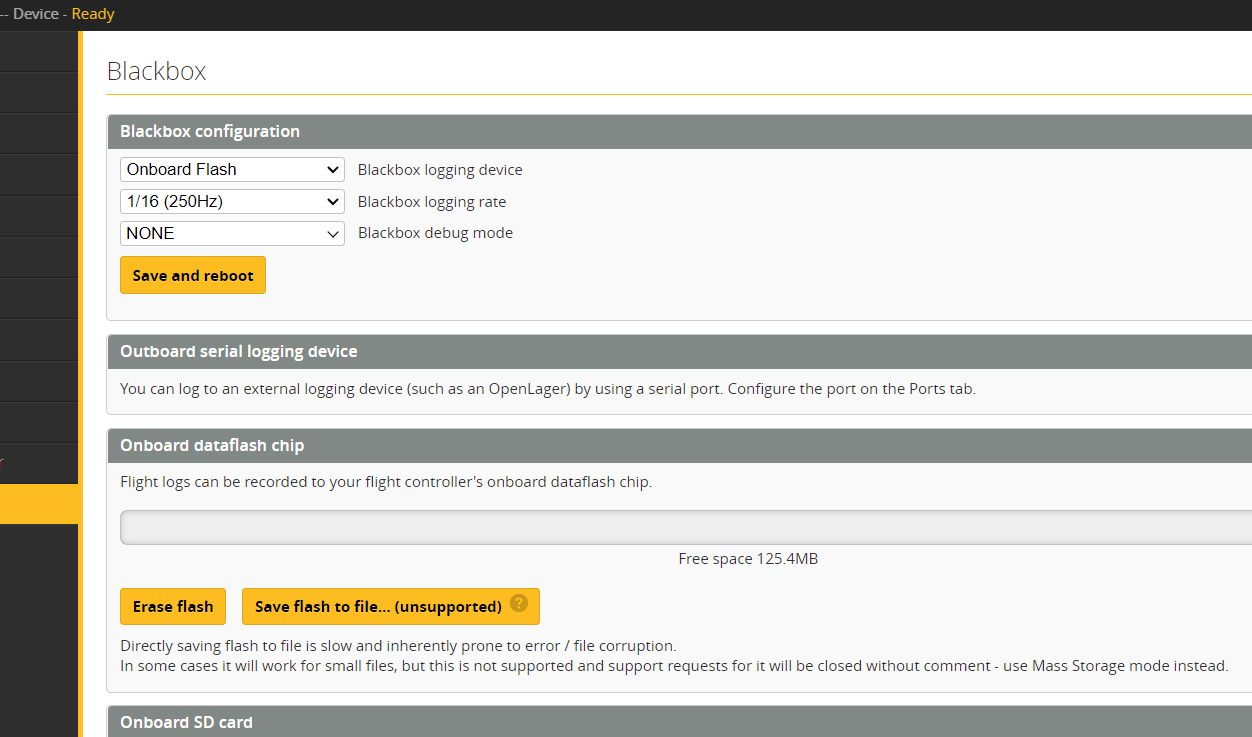The interface features a black border at the top, with "Device Ready" inscribed on the left. A dark gray border on the left is intersected by a yellow horizontal line. Adjacent to this, a white box on the right displays "Black Box," below which a yellow line runs horizontally. Beneath that, a gray box labeled "Black Box Configuration" in white text is present.

Below the "Black Box Configuration" section, a dropdown menu labeled "Onboard Flash" appears, accompanied by the text "Black Box Logging Device." Further down, another dropdown menu shows "116, 250 Hz," adjacent to "Black Box Logging Rate." Beneath this is a dropdown menu labeled "None," with "Black Box Debug Mode" to its right. Following this is a yellow rectangular button marked "Save and Reboot."

A light gray line then stretches horizontally across the interface, beneath which lies a dark gray box labeled "Outboard Serial Logging Device" in white letters. Below this, the text explains: "You can log to an external logging device such as OpenLogger by using the serial port. Configure the port on the Ports tab." Lastly, a dark gray box at the bottom reads "Onboard Data Flash Chip."